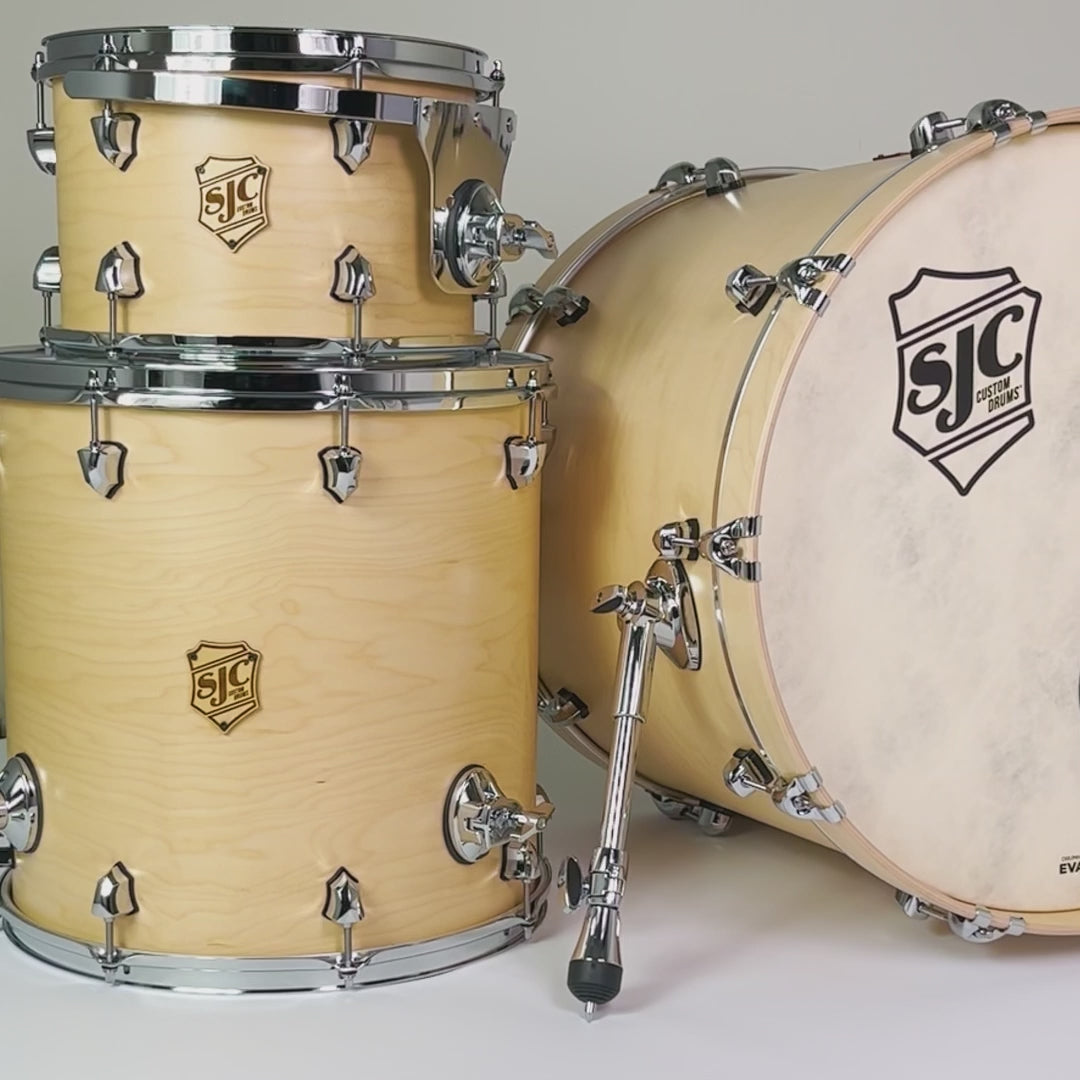A high-quality drum set is meticulously arranged on a pristine white surface against a seamless white background, akin to a studio photography setup. The central focus is on the natural wooden finish of the drums, showcasing a light wood color highlighted by elegant brown wood grains. On the right side of the image, partially cut off, is the prominent bass drum, identifiable by its horizontal position and the pedal mechanism. This drum features numerous metal brackets around its body, enhancing its robust appearance. The drumhead, made from thick, leathery material, prominently displays the SJC Custom Drums logo, shaped like a shield, adding a touch of prestige.

To the left of the bass drum, a stack of two smaller drums is neatly aligned. The larger of the two sits at the bottom, with a smaller drum perched on top. Both drums share the same natural wooden aesthetics and are adorned with chrome frames and brackets, providing a striking contrast. Each drum proudly bears the SJC shield logo, confirming their custom craftsmanship and cohesive design. The overall arrangement and presentation emphasize the superior quality and craftsmanship of these drums, making them a centerpiece in any musical setup.